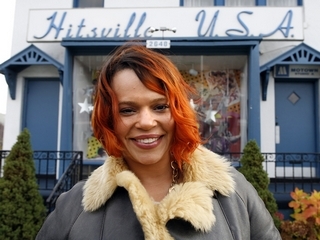In this vibrant photo, Faith Evans stands confidently before the iconic Motown Museum, famously known as "Hitsville, USA." Dressed for cooler weather, she dons a cozy, puffy gray jacket adorned with a light brown fur collar and lining, which complements her striking reddish-orange hair with visible dark roots. Faith’s warm smile, revealing her top row of teeth, radiates towards the camera.

The background captures the festive essence of the season, with stars hanging across the museum's window, hinting at a holiday atmosphere. An evergreen tree stands tall on the left, while subtle decorations adorn the right, evoking the spirit of Christmas. The museum itself, with its distinctive blue and white facade, features white-trimmed doors on either side and a small black iron railing in front. A bush with brown leaves adds a natural touch to the scene, enhancing the overall warm and inviting feel of this snapshot.